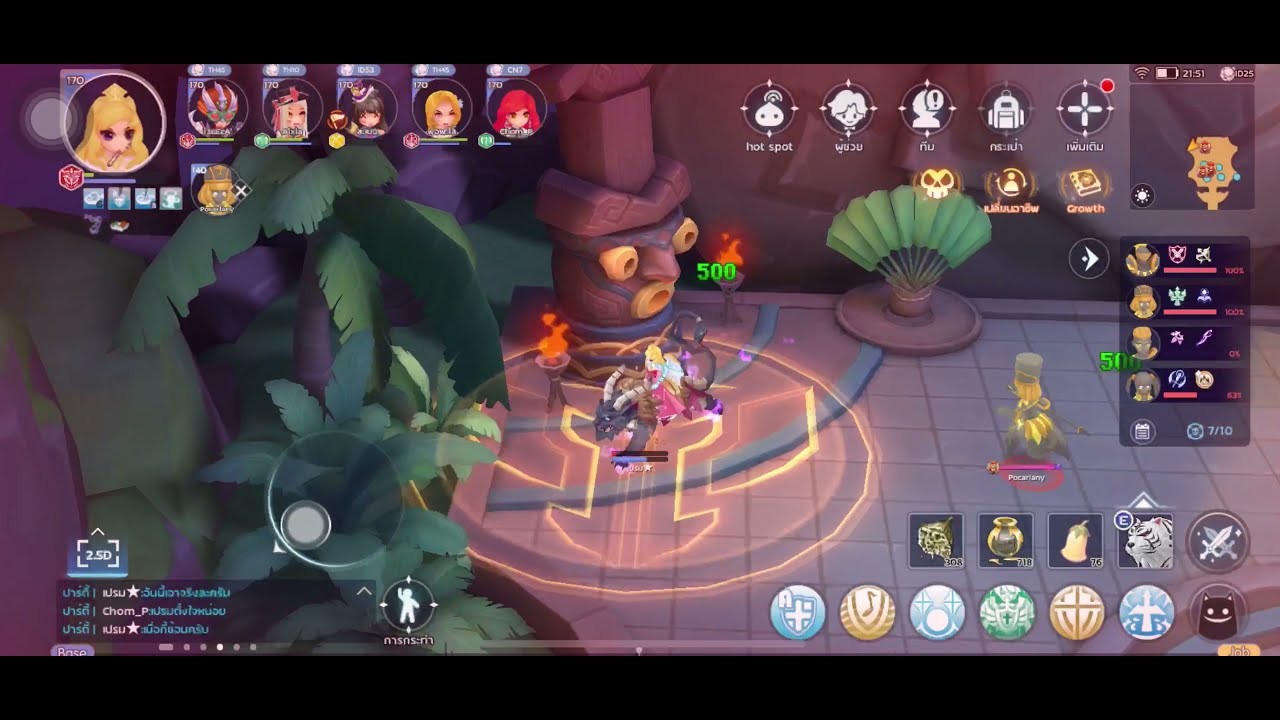This screenshot from a video game captures a dynamic and colorful scene. The main focus is a female character with blonde hair, donning a pink dress, who is riding a gray beast with white horns. This character is slightly off-center to the left, indicating she might be controlled by the player. Surrounding her, the environment is filled with various vibrant elements such as green plants and trees, which resemble palm trees or decorative elements like a Chinese fan in a pot. The ground appears to be tiled with a dark red and yellow color scheme.

To the right of the main character, there is a ghost-like figure, also seemingly controlled by another player. The upper left corner of the screen showcases a series of player icons, which include different characters with diverse appearances such as blondes, redheads, and brunettes. The top right corner contains more icons, some of which resemble a clay pot and crossed swords. The bottom right corner features a selection of sticker emblems and game control icons, including options like a cross and a musical note. There's also a chat box in the bottom left displaying text in a different language, with a visible sticker saying "Hotspot" and the numeral "500" repeating in the score display. 

Overall, the scene portrays a bustling and richly detailed video game environment with a focus on interactive elements and user interface components, blending various colors and characters seamlessly.